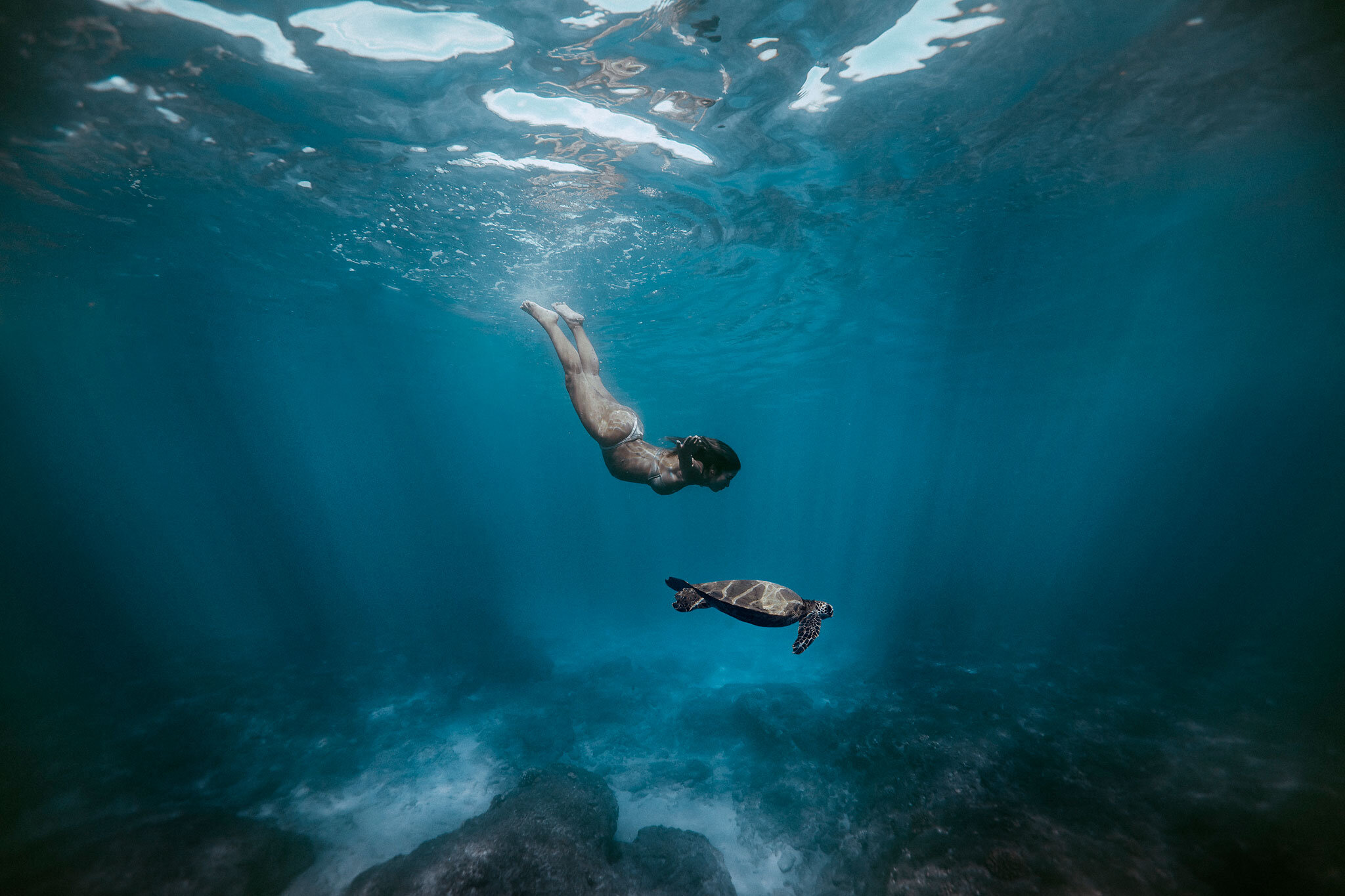In this underwater photograph, a brunette woman in a white bikini is captured diving gracefully downwards, her body fully immersed just below the surface. Her arms are extended to her sides as she gazes intently at a brown sea turtle swimming directly beneath her. The water surrounding them is a vibrant mix of deep turquoise and cyan, with sunlight filtering through, casting intricate patterns of light and shadow that dance across both the woman and the turtle. The bottom of the image showcases a seafloor speckled with white sand and black rocks. Behind this serene moment, the expansive, crystal-clear water extends into the background, creating a stunningly vibrant tableau. The reflective surface of the water above them hints at the world above, adding a magical, almost ethereal quality to the scene.